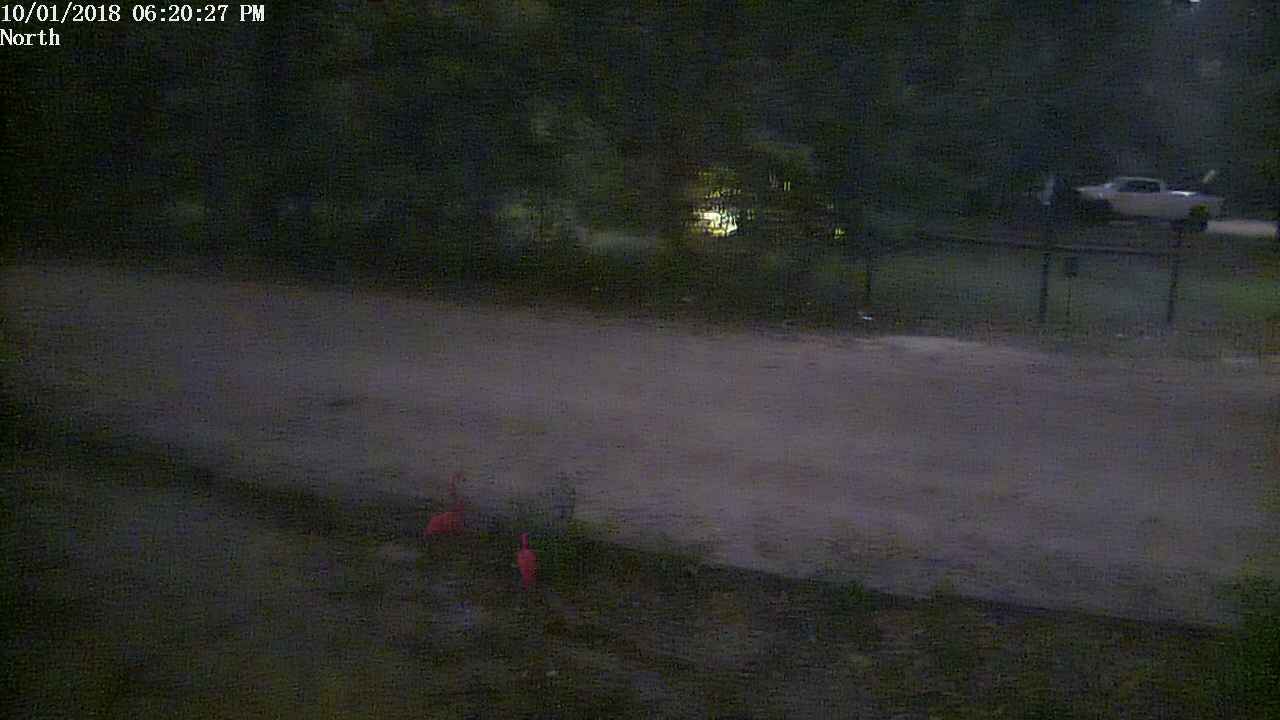In this grainy, out-of-focus image, a small flock of flamingos stands gracefully beside a road. In the foreground, a fence runs parallel to the road, partially obscured by some foliage and, faintly visible in the distance, a light. To the top right of the image, a white truck is parked on a driveway, positioned towards the left from this perspective. The background features a field of grass, adding to the natural setting, but no other animals or distinctive elements are discernible in this dimly lit, hazy photograph.